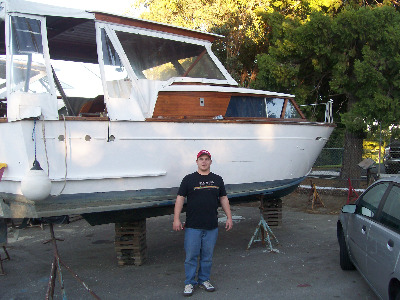In the daytime outdoor scene, a man poses in front of a white cabin cruiser boat propped up on cement tiles in a boat yard or possibly a backyard. The boat, which appears to be undergoing renovations, features wood paneling, a glass cabin, and fabric protection on top. The man, dressed in blue jeans, sneakers, a black t-shirt with yellow writing, and a red baseball cap, stands confidently in front of the boat. To the right, a gray, four-door sedan is parked near the vessel. The background reveals a fence and a line of mature trees, with the boat resting on an asphalt surface scattered with cones. The setting combines elements of a working environment and a casual, everyday atmosphere.